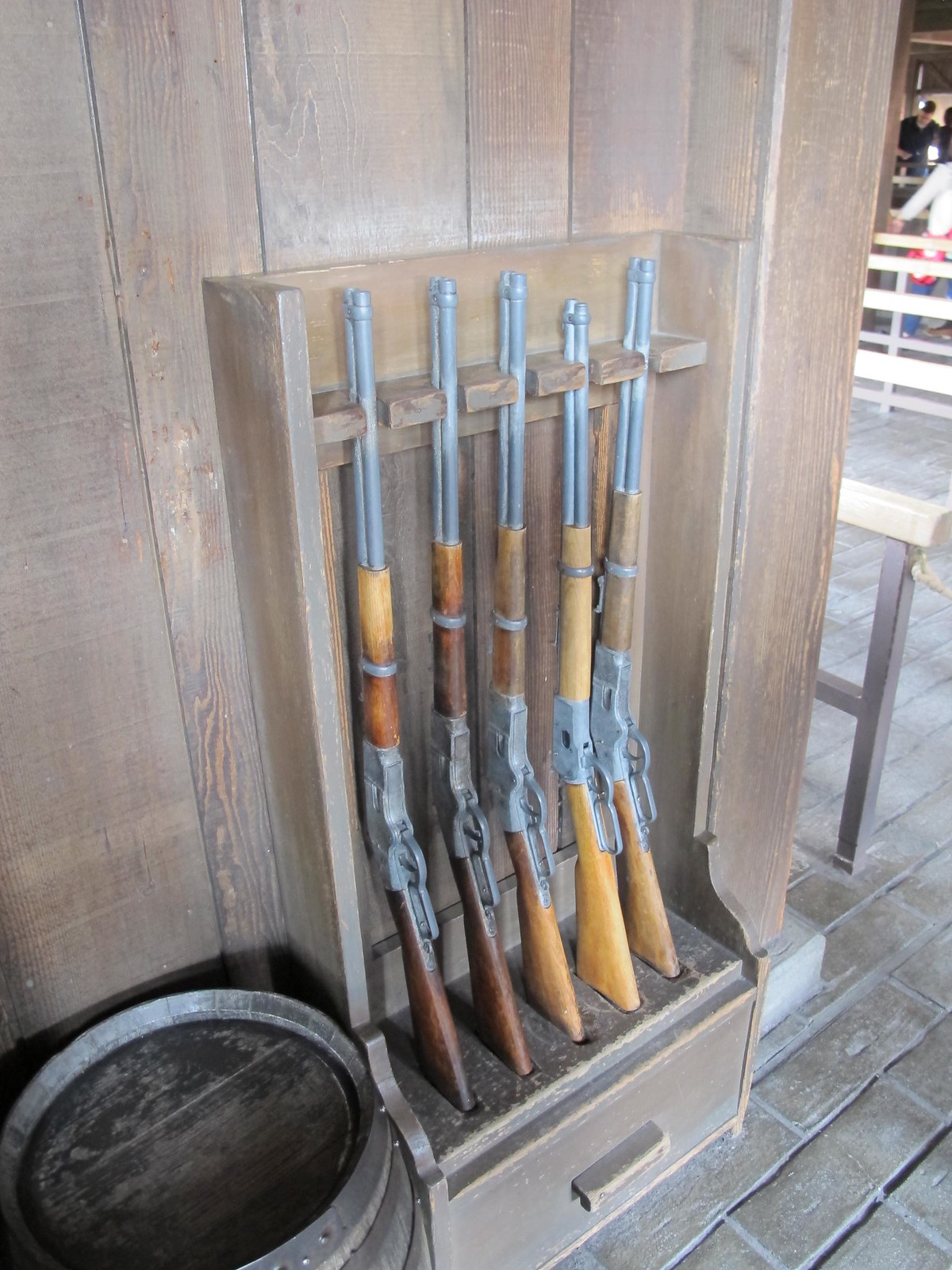The photograph showcases a vertical gun cabinet made of dark stained wood, positioned against a wooden wall, with a drawer beneath it featuring a wooden handle. Inside the cabinet, five lever-action rifles are neatly arranged, each resting butt-down in individual slots and secured at the top by notches. The rifles share a uniform design characterized by wooden stocks and hand grips, varying in shades of brown, and tarnished silver metallic components that suggest extensive use. The barrels of the rifles are a dark silver-gray, reflecting their well-used nature. To the left of the cabinet, a worn, dark wooden barrel is partially visible, while on the right side, a faint glimpse of a person behind a fence can be detected. The floor beneath is composed of faded reddish-brown brickwork.